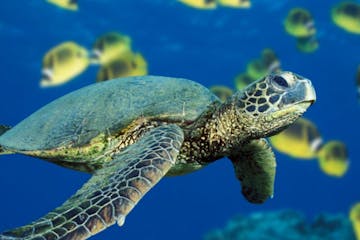This vibrant and detailed underwater photograph captures a medium-sized sea turtle swimming gracefully in a deep, vivid blue ocean. The turtle occupies the majority of the foreground and appears to be gazing toward the viewer with its oval-shaped eyes. The turtle's shell is a striking green, contrasting with its blue-gray skin and rough-textured neck. The shell's unique patterns and scales are prominently visible, adding to the turtle's majestic appearance. Surrounding the turtle, a school of green and yellow tropical fish can be seen, their white-ringed tails and striped bodies weaving in and out of the frame. The fish are slightly out of focus, giving depth to the image. In the bottom right corner, a part of a coral or stone formation is faintly visible, grounding the scene in the underwater landscape. This serene and picturesque moment captures the peaceful cohabitation of the turtle and fish in their natural, undisturbed aquatic habitat.